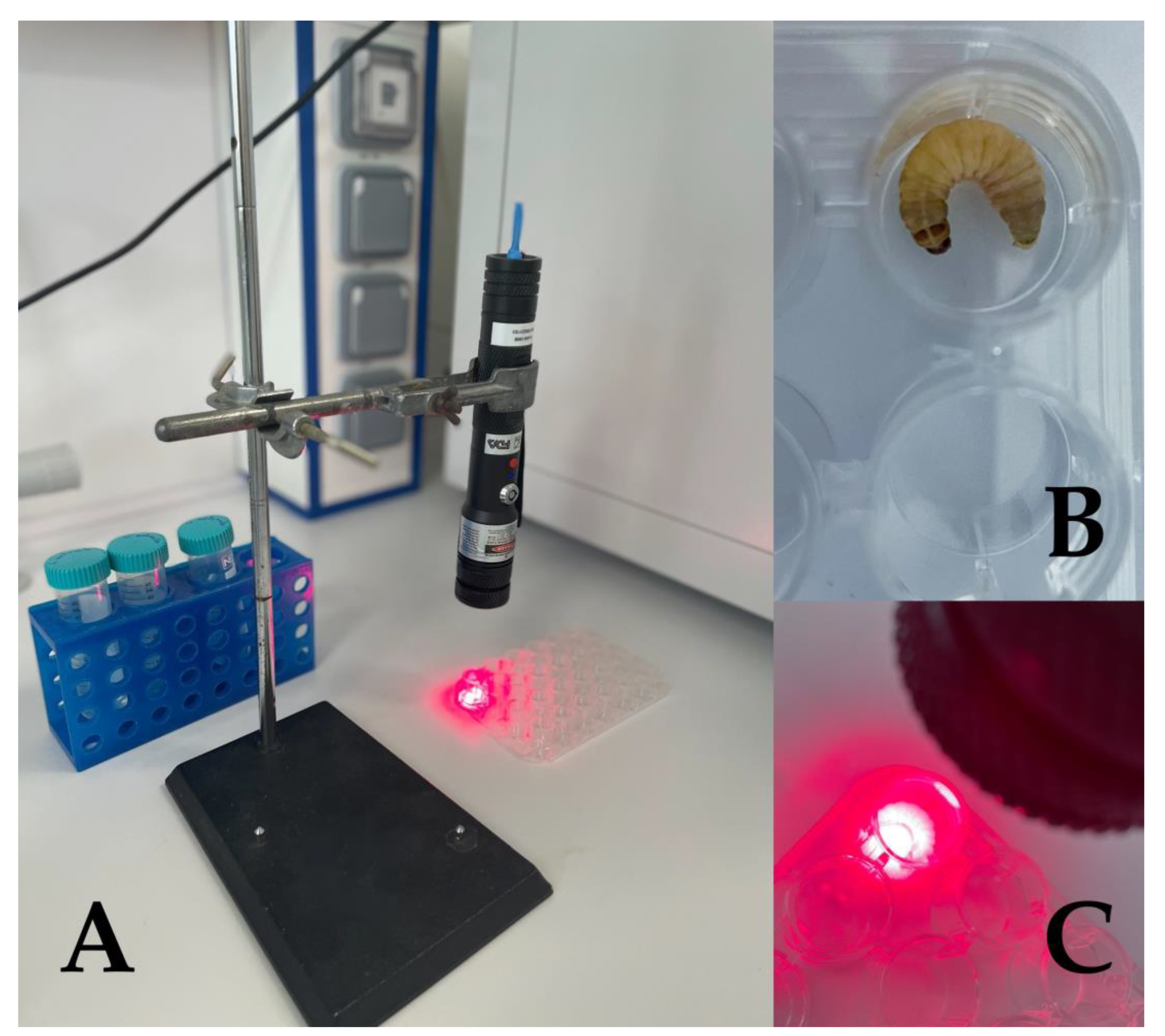The image consists of three photographs, arranged side by side. The left photograph, labeled "A" in the bottom right corner, captures a laboratory setup featuring a microscope or laser apparatus. This device is mounted on a black stand with a metal arm that holds a light source emitting a pink-hued beam. This pink light transitions from white to deep pink and is directed onto a small tray beneath. Adjacent to this setup is a blue plastic holder containing several vials with blue caps.

The top right photograph, labeled "B" in the bottom right corner, provides a close-up view of the tray, revealing a light tan worm or larvae within it. The bottom right photograph, labeled "C," offers another close-up focused on the same pink light shining onto the tray, making the worm visible. Together, these images depict a detailed scene of a scientific examination or experiment involving a light source, possibly a laser, highlighting the subject within the tray.